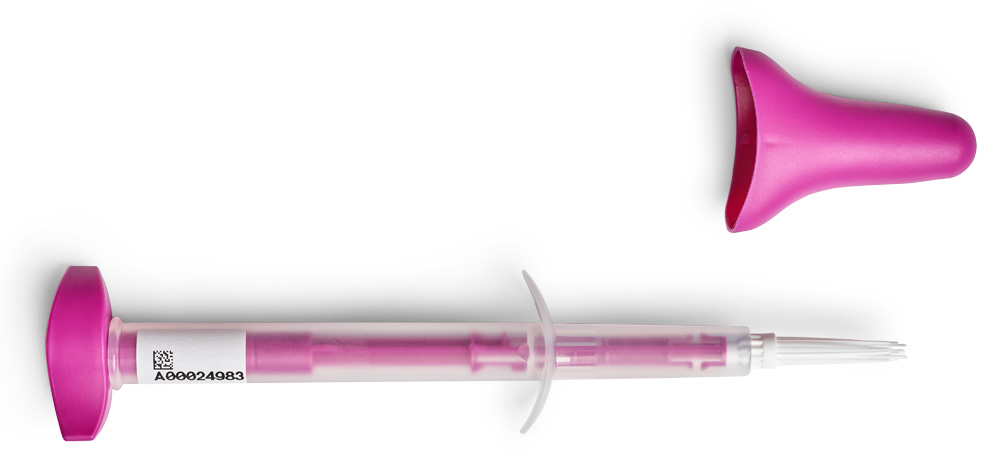The image features a medical device, positioned horizontally, against a white background. In the top row, to the right, is the cap of the device, which is a slightly darker variant of hot pink. The cap has a conical shape: its opening faces left, and the pointed end faces right. Below the cap, in the bottom row, is the main body of the device resembling a needle or dropper. This cylindrical component is made of clear plastic, housing a bright pink plunger inside a purple chamber. The device also has a white, pointed tip on the right end, and a guard or handle on the left side. The handle includes a QR code and the label "A00024983" in black font. Midway along the device, clear plastic wings or fan grips add to its functional design, enhancing usability.